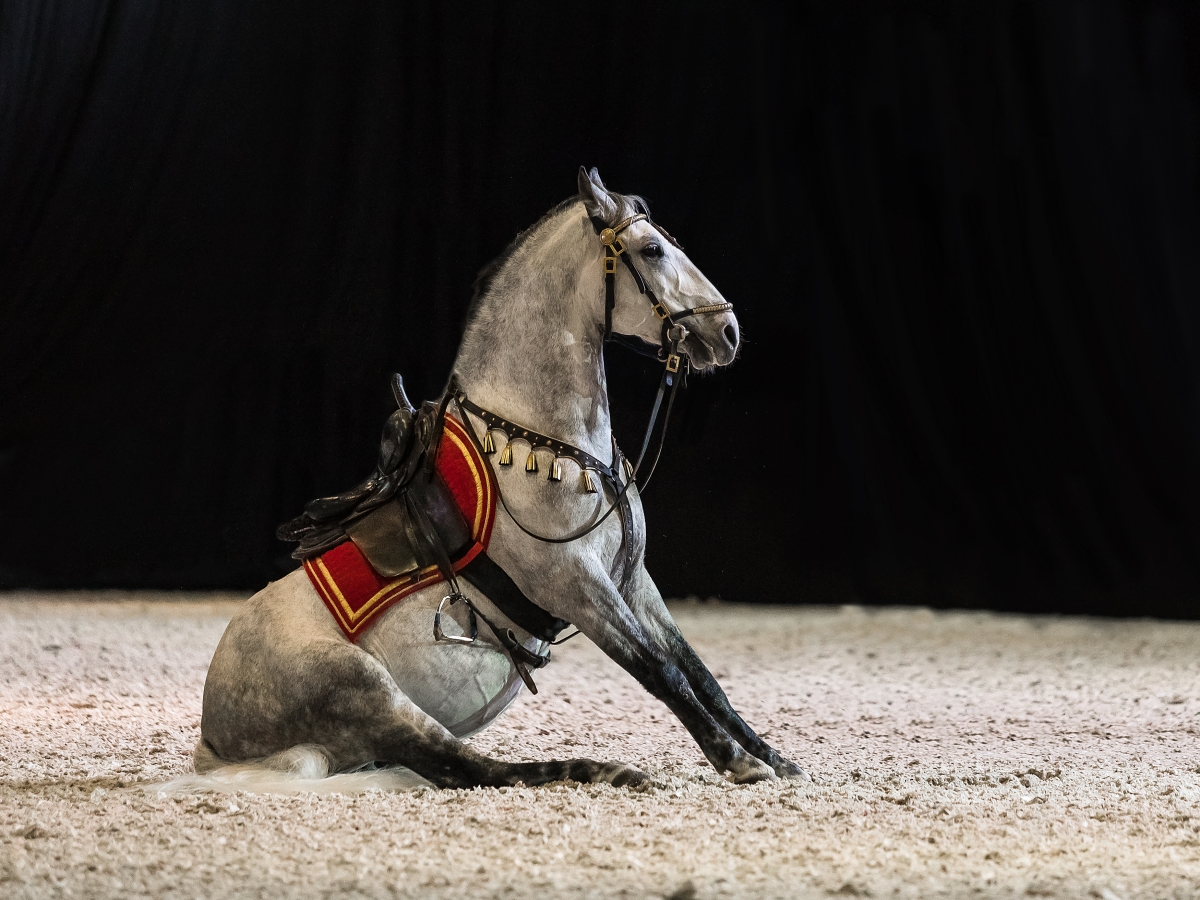The photograph centers on a white horse with grayish and black markings, seated on a beige gravel surface. The horse's posture suggests he is sitting on his haunches with his front legs extended forward to support his body, creating an unusual and almost human-like sitting position. The horse is fully equipped with a black leather saddle and a red padded blanket underneath, which is adorned with gold accents. The reins and the belt that circles his body are black with gold ends, and gold clips can be seen near the harness around his ears. His ears are perked up, adding to his alert appearance. The lower part of his legs appears darker, almost black, against the predominantly white fur. The background is entirely dark, emphasizing the horse and the gravel he sits on. The photograph's lighting distinctly illuminates the horse from the right side, enhancing the textures and details of his coat and equipment.